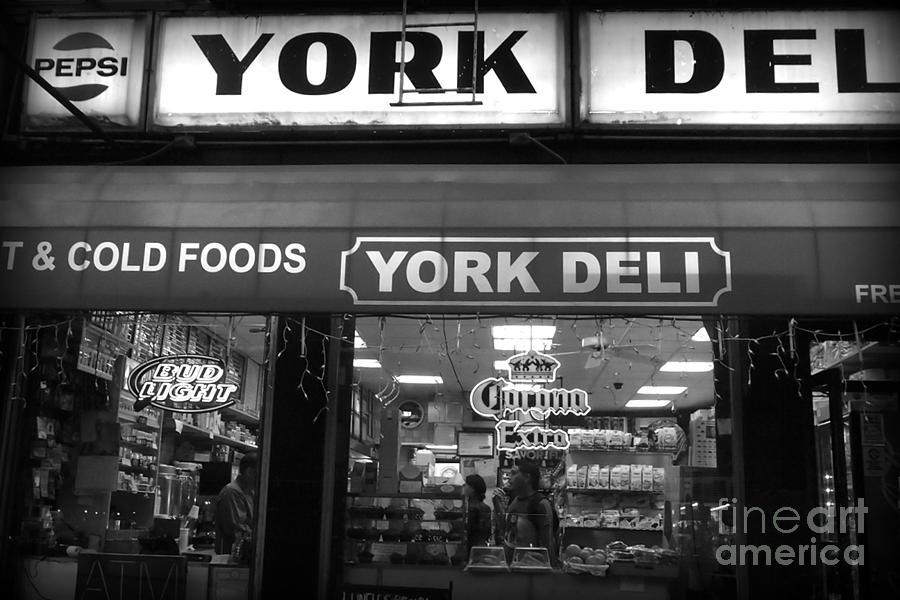This black and white photograph captures the striking facade of York Deli, an old-fashioned store with distinct signage and bustling activity inside. The top left corner features a square neon Pepsi sign, while adjacent to it are two rectangular illuminated signs reading "York" and "D-E-L," short for "Deli." Beneath these signs is an awning displaying "Hot and Cold Foods" alongside "York Deli" in bright white text. Large glass windows dominate the front, showcasing the lively interior where a cash register is visible to the left and people, along with various food items, occupy the right side of the image. Notable details include neon window ads for Bud Light on the left and Corona Extra on the right. The store's interior brims with products like oranges, bread, muffins, and a cake under glass, while a person works behind the counter. In the lower right-hand corner, the photo is marked with "Fine Art America," suggesting its artistic value. This richly detailed snapshot encapsulates a moment in time at a traditional deli, rendered in monochromatic tones.